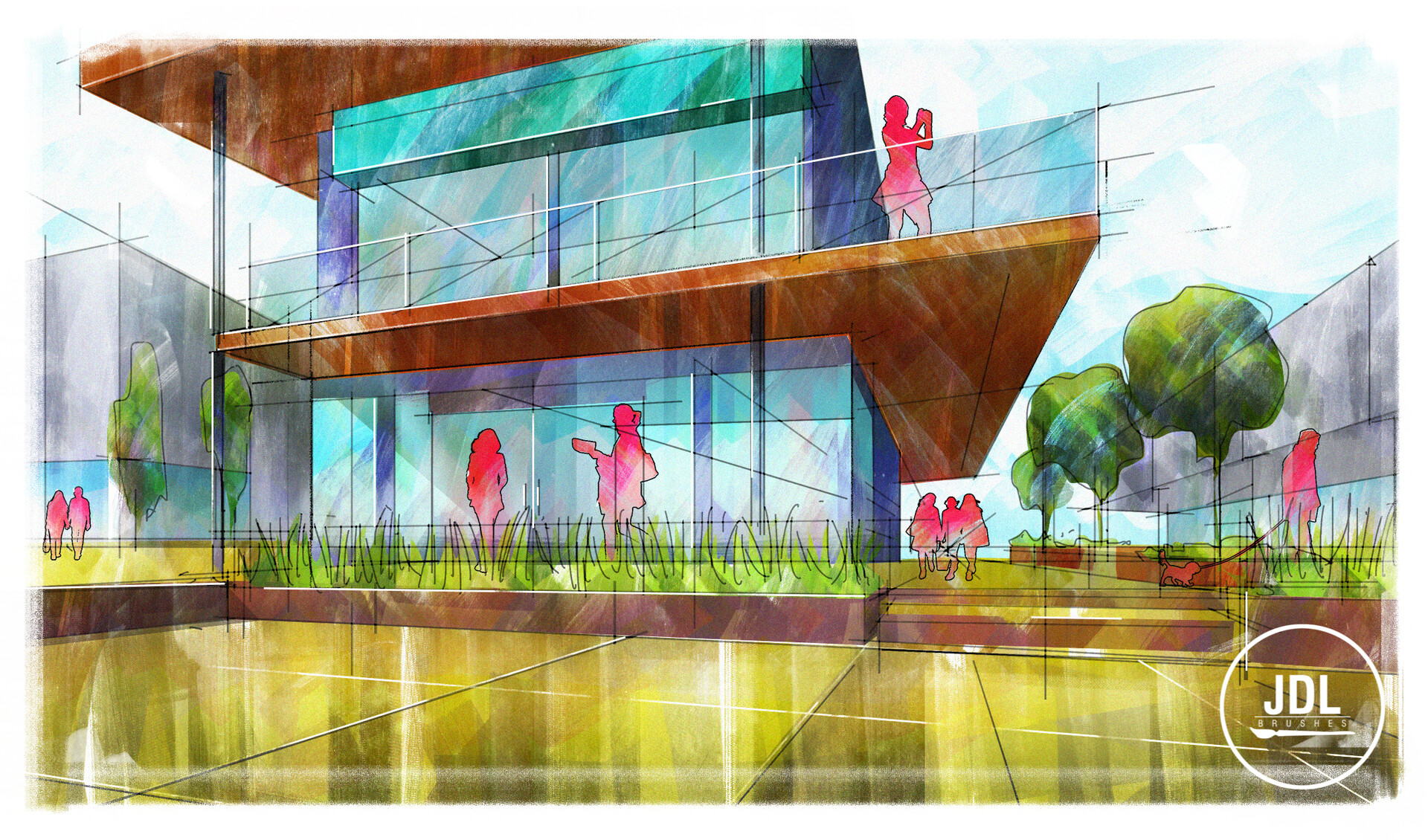The image depicts a detailed architectural drawing of a sleek, futuristic two-story glass building, prominently centered within the frame. Created using a digital medium, possibly AI-generated or painted, it exhibits modern design with a mix of materials including glass and wood. The ground in the foreground is a yellow cement patio, with visible impressions where the boards were placed during its construction. There's a slightly elevated sidewalk to the right, accompanied by planters containing representative greenery.

The building itself features a wood deck that extends outwards, forming a balcony on the front and right side. The roof, characterized by a brown hue, extends over to the left and is supported by a pole. Scattered throughout the image are figures depicted in vibrant red, adding a lively touch to the scene—one notable figure is a lady standing on the upper level holding an object. 

The image's color palette includes blue, green, pink, white, brown, and gray, contributing to its modern and clean aesthetic. The environment hints at a futuristic cityscape, with additional buildings and trees to the right of the main structure. In the bottom right corner, a white circle displays the inscription "JDL Precious," marking the artwork with the creator's signature.